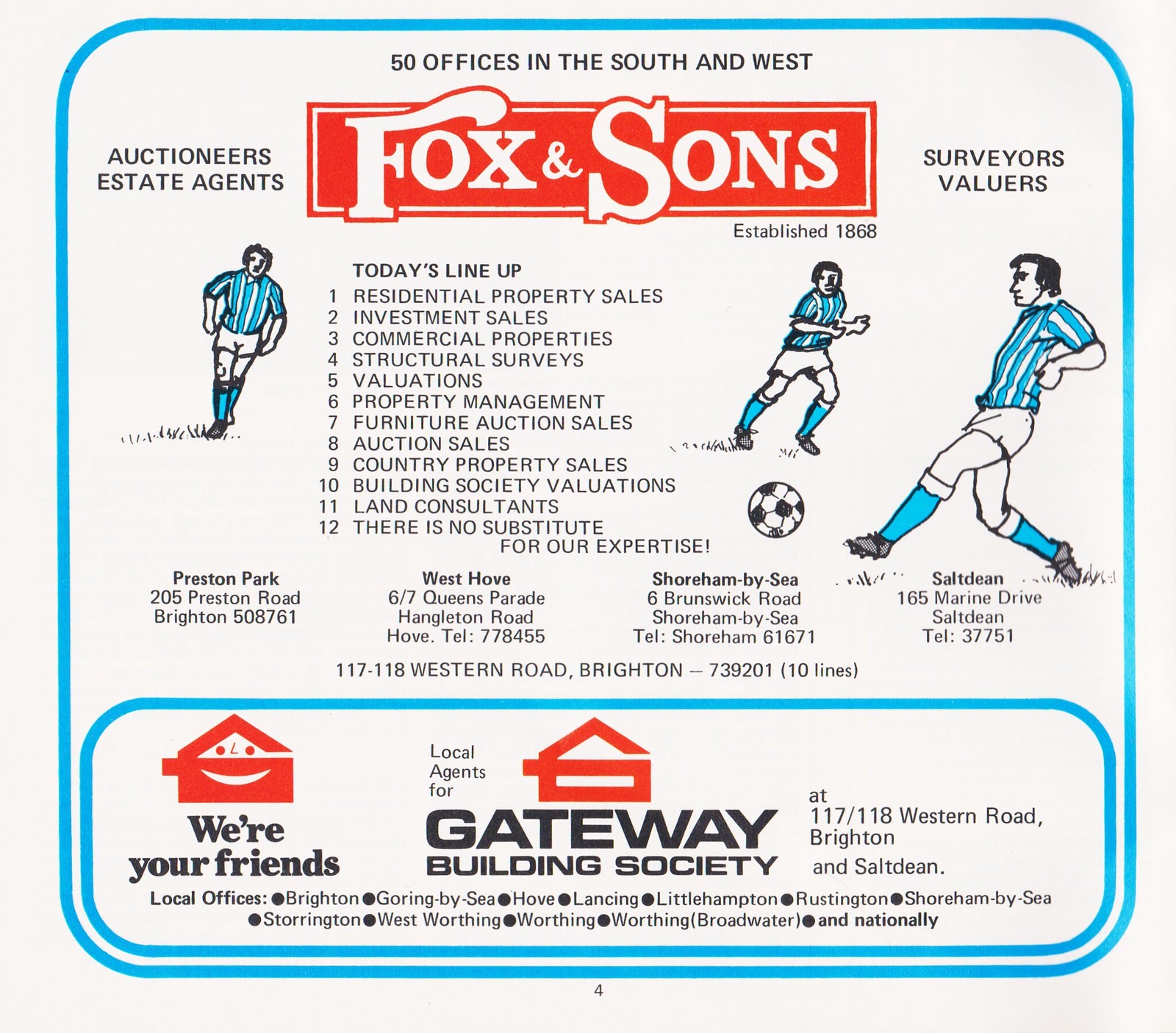This image, likely a newspaper or magazine advertisement for Fox and Sons, established in 1868, showcases their comprehensive services and local expertise. The ad is set on a design featuring a blue outline with a white center, and black lettering highlighting "50 offices in the South and West." A prominent red rectangle serves as a backdrop for the brand's name, emphasizing their long-standing reputation as surveyors, valuers, auctioneers, and estate agents. Detailed listings under "Today's Lineup" include residential property sales, investment sales, commercial properties, structural surveys, valuations, property management, furniture auction sales, country property sales, and land consultations, all underscored by the statement "There is no substitute for our expertise." An illustration within the ad shows three people in blue and white uniforms playing soccer, linking to the community-driven spirit. Locations mentioned include Brightington, Hove, Shoreham, and another local office, all collaborating with the Gateway Building Society, reinforcing their commitment as local agents.